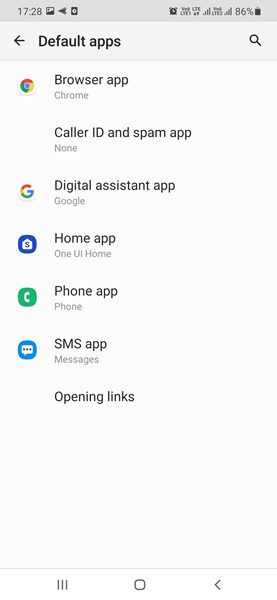This is a detailed screenshot of a smartphone screen displaying the default apps settings in a light gray interface. The top banner is light gray with a timestamp of 17:28, accompanied by several icons: a photos icon, a left-facing send icon, an indistinguishable black icon, a clock icon, an LTE signal indicator, a battery at 86%, and a Wi-Fi indicator.

Below the banner, a lighter gray section contains a left-facing black arrow with the text "Default Apps" to its right and a search box below it. The settings are listed in vertical order:

1. **Google Logo** - "Browser app" set to Chrome.
2. **Call ID and spam app** - None.
3. **Google Logo** - "Digital assistant app" set to Google.
4. **Money Icon** - "Home app" set to One UI Home.
5. **Phone Icon** - "Phone app" set to Phone.
6. **Comment/Message Box Logo** - "SMS app."

Further down, a section labeled "Opening links" is visible. The bottom border of the screen is white, featuring several navigation icons: a drop page icon, three vertical dots, a home button, and a left-facing arrow.